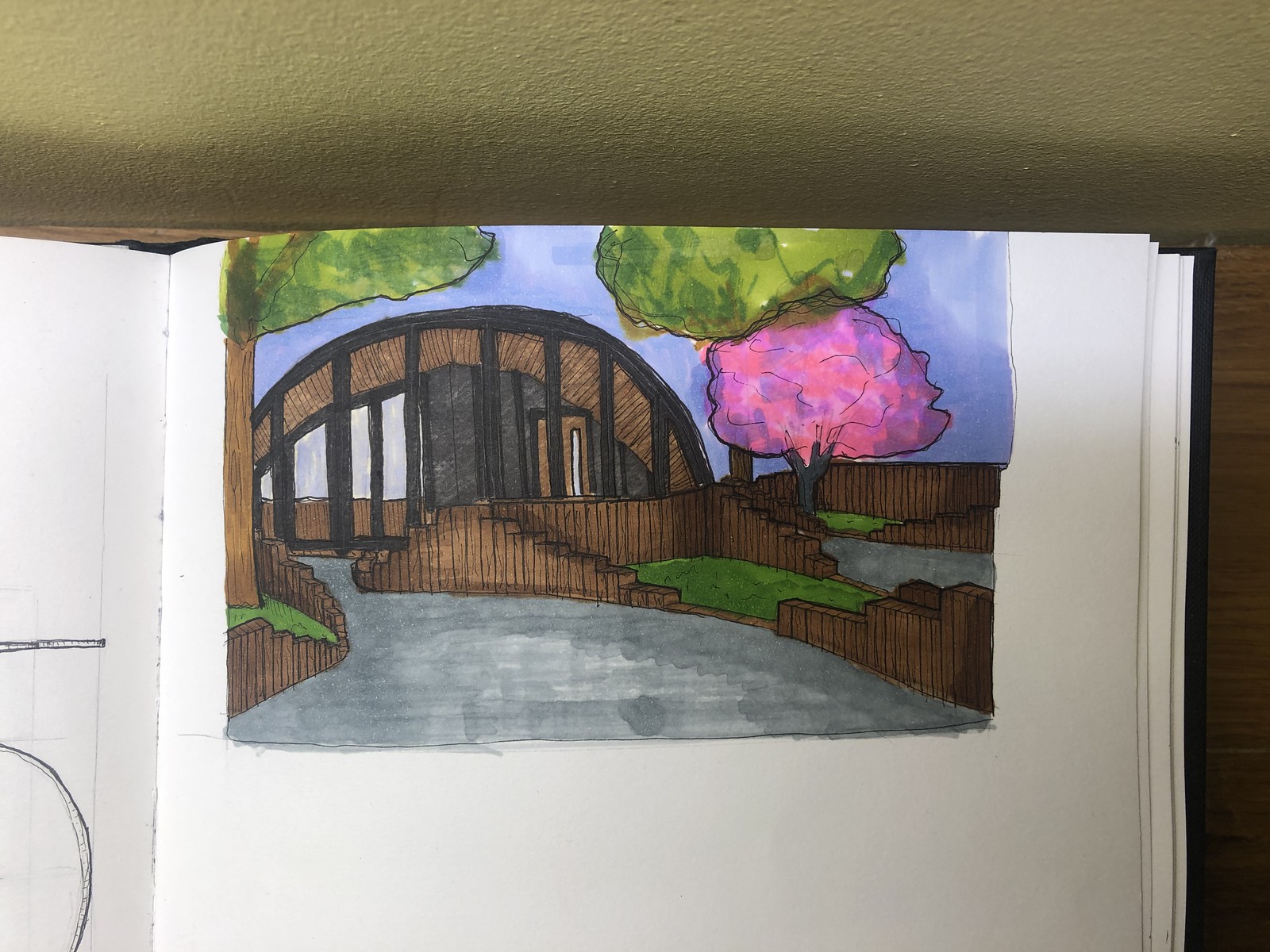The image depicts a scene with various elements artfully arranged. The ceiling appears rough in texture, adding an element of rustic charm to the overall composition. On the right-hand side of the image, an open notebook is prominently positioned. The notebook contains sheets of paper—some covered in linear patterns. The left side of the notebook features a detailed watercolor painting. 

In this painting, a tall tree with a vivid green canopy, resembling a bush perched atop its trunk, dominates the left side. To the right, another tree stands out with a mix of lighter and darker green leaves, adding depth and variation to the greenery. Additionally, there's a striking pink tree, adorned with hints of purple, contributing a whimsical touch to the display.

Framing the scene are brown walls, which contrast with sections of green and gray hues, providing a layered backdrop. An archway is visible in the background, offering a glimpse into another space and enhancing the scene's intricate detail and depth.